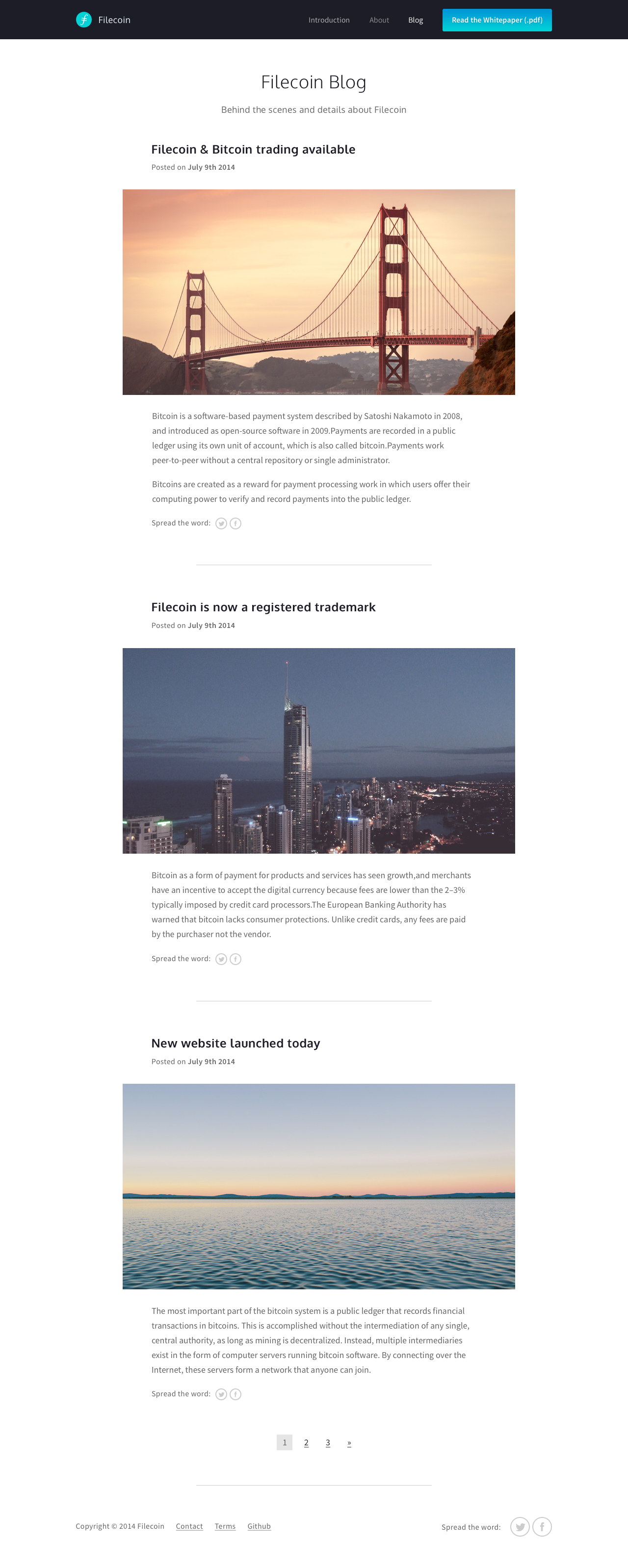The image features a composition with several distinct elements. At the top, a black bar contains text that is too blurry to decipher. On the left side, there is a teal-colored circle, which is mirrored by a teal bar on the right. Below this header, the words "something blog" can be seen, followed by some more illegible text. 

Central to the image is a pixelated and grainy photograph of what appears to be the Golden Gate Bridge, characterized by its iconic suspension design, flanked by mountains on both sides and a body of water beneath it. The bridge is depicted in an orange-copper hue. Below this image is a paragraph of text.

Further down, bold text introduces a new section, accompanied by an image of a city skyline at either nighttime, dusk, or dawn, featuring a building prominently in the foreground. Another paragraph of text is placed below this skyline image.

Towards the bottom of the composition, a new bold header leads into an image showing an expansive ocean, a blue sky, and a bright orange horizon, possibly depicting either sunrise or sunset. A final blurry paragraph of text rounds off the image at the bottom.